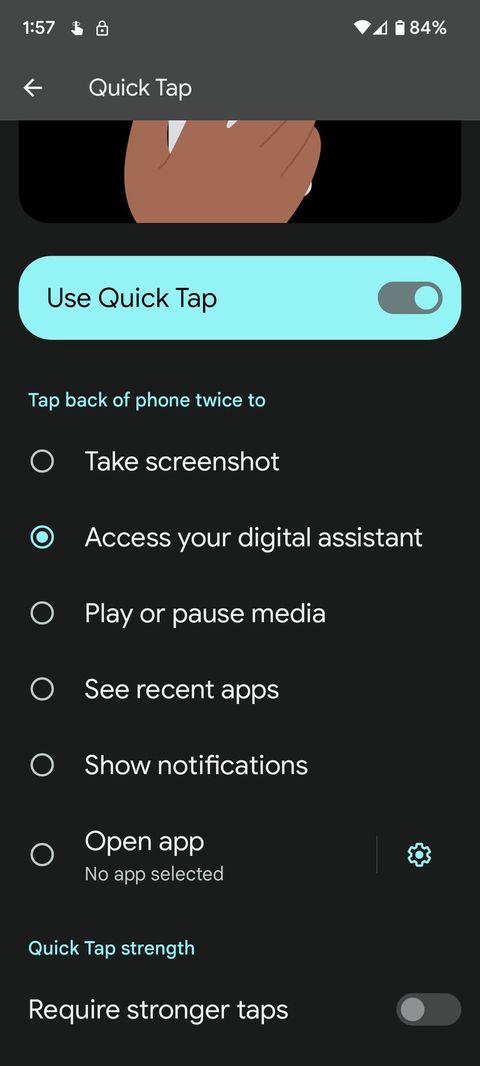This is a detailed screenshot of a phone interface. The top 2 inches of the screen features a dark grey background. In the top-left corner, the number "157" is displayed, followed by an icon of a hand with the index finger pointing up and the thumb oriented to the right, while the other fingers are curled down. To the right of this hand icon is a white outline of a lock icon. Further to the right, the battery percentage reads "84%", accompanied by a nearly empty white battery icon next to it. Adjacent to the battery icon, there is an internet icon that is half-filled white, with the other half grey, followed by a fully-filled WiFi signal icon. 

Directly below the number "157" is a white arrow pointing to the left, next to the text "Quick Tap" in white. Underneath this, there are small grey tabs on both the left and right sides, and a central black box about an inch in height featuring an outline of a cartoon-like hand.

Below this, a large rectangle with rounded edges spans the width of the screen. This rectangle is teal-colored and contains the words "Quick Tap, Use Quick Tap" in black. Inside this rectangle, a smaller grey tab is positioned, with a blue circle on the right side indicating that it is toggled on. 

Beneath this section, small blue text reads, "Tap back of phone twice to," followed by a vertical list of circular icons with white outlines. The second circle from the top has a blue button in the middle, indicating it is active. Six options describe the actions that tapping twice will execute, with the final item reading "No app selected." 

To the right of the bottom option, an icon resembling a settings gear is displayed. Below this, small blue text reads "Quick Tap strength," followed by a description, "Require stronger taps," with its corresponding toggle set to off.